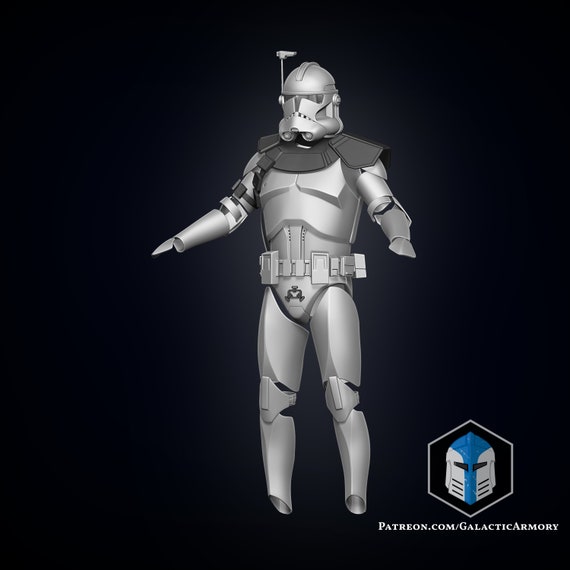The image showcases a detailed 3D rendering of an armor suit designed in the style of a Stormtrooper from Star Wars. The suit, seemingly devoid of a wearer, stands centered against a stark black background. The primarily white armor is accentuated by various shades of gray, including dark gray segments around the shoulders. The suit comprises several components: a helmet with an integrated mask, shoulder armor, and a main body piece, all connected by a belt around the waist. Notably, the armor lacks hands and feet, giving it an unfinished appearance that could be intended for 3D printing purposes. Additionally, an intriguing feature protrudes from the right side of the helmet, resembling a tracking beam or laser device. In the bottom right corner, a logo featuring a helmet with a blue stripe and encased in a hexagonal gray border is visible, accompanied by the text "Patreon.com/GalacticArmory" in white font, indicating a connection to the Galactic Armory's store or promotional material.